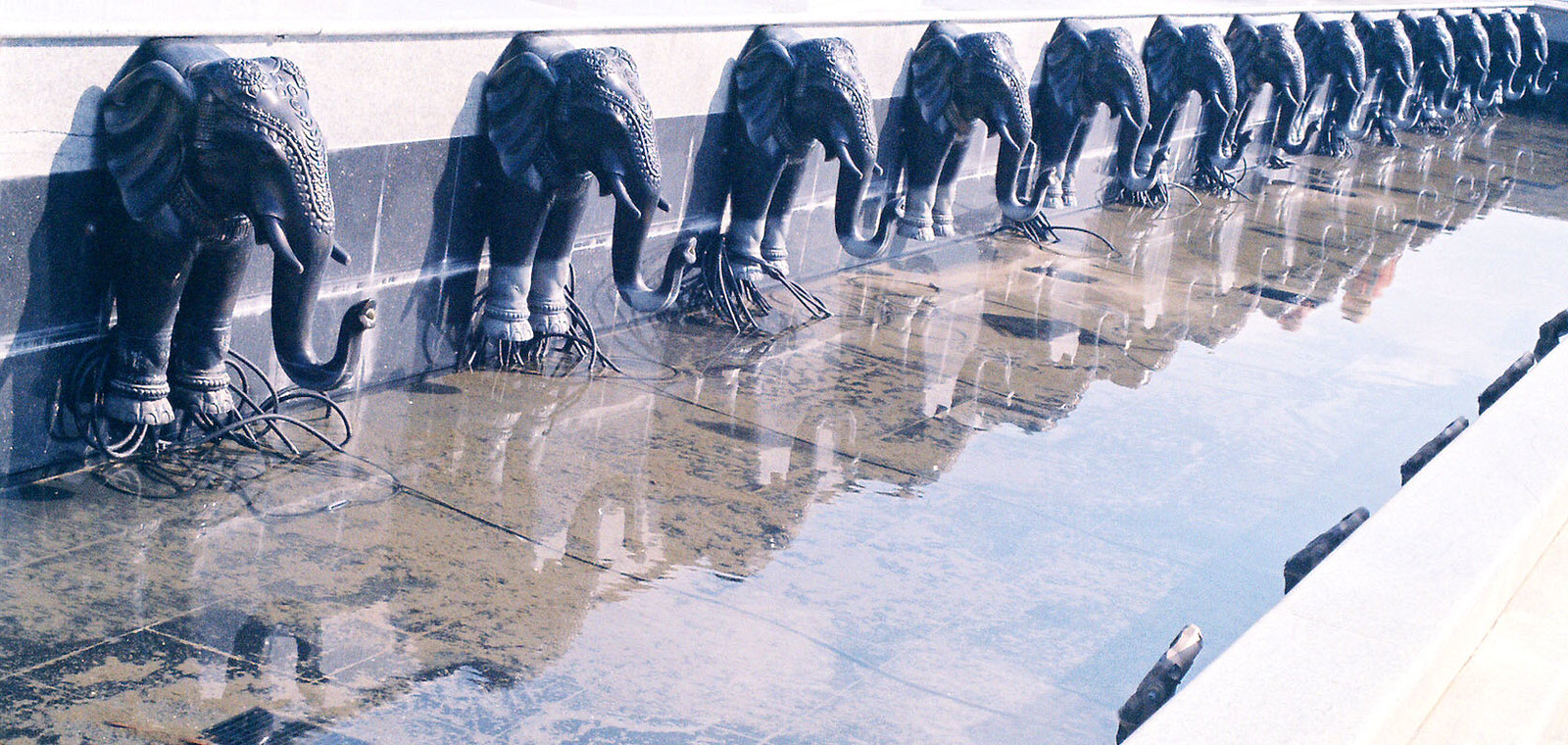The image depicts a partially drained, shallow water fountain or moat lined with intricately designed gray elephant statues. These statues, each featuring tusks and engraved details around their faces and ears, extend from the left to the right corner of the gray and white grouted wall they are affixed to. Visible are the front two legs, ears, face, and trunks of 13 elephants, and most have black tubes or cables near their feet, suggesting a system for siphoning or spraying water. The water level is shallow enough to see the ground beneath, indicating it might be in the process of draining. The wall behind the statues features alternating stripes of gray and white, reflecting off the wet surface below.